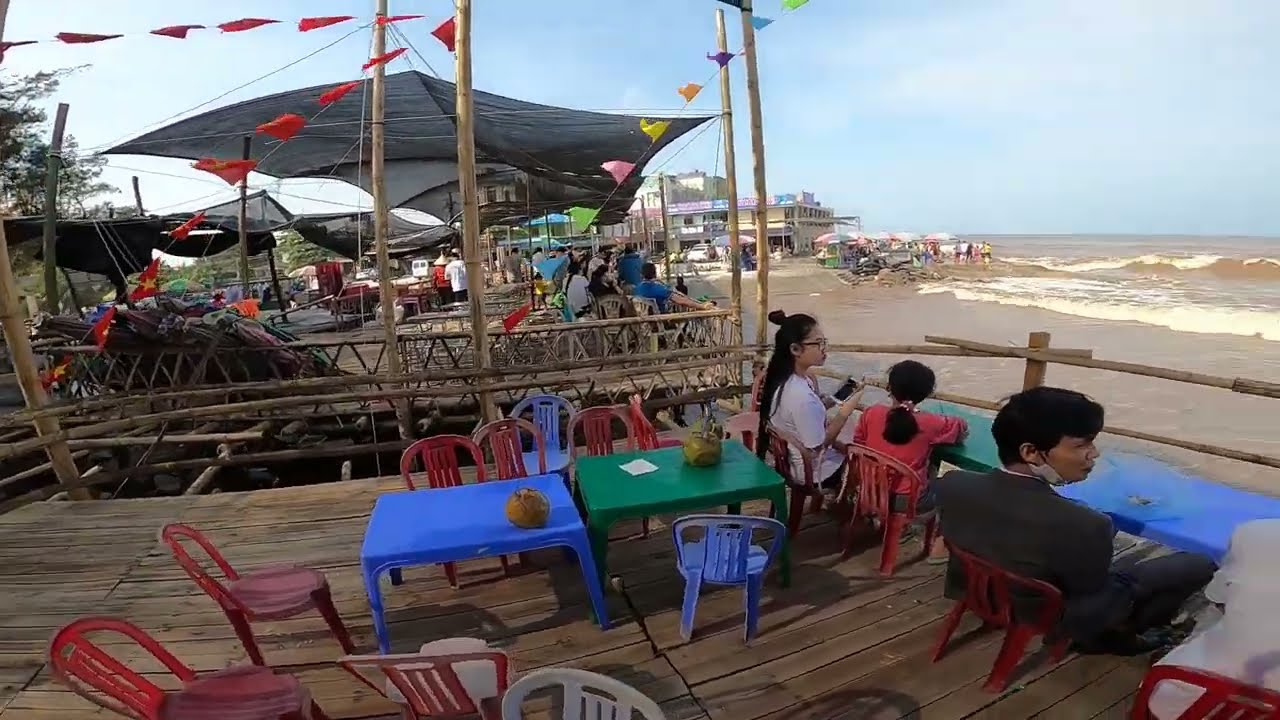The photograph captures a group of four people—two young girls, an adult man, and an adult woman—relaxing on a bamboo and wooden deck that extends from an outdoor bar restaurant. The deck, located by a muddy, brown beach, is furnished with blue and green plastic tables, and various colored lawn chairs in red, blue, green, and white. The man is dressed in a grey shirt and blue jeans, with a face mask pulled down, while the young girl next to him wears a red long-sleeve shirt and blue jeans, her hair pulled back into a ponytail. Another girl in a white t-shirt sits beside her, and across from them is a person wearing another white t-shirt. 

Scattered around are multiple closed umbrellas and awnings, which offer minimal shade. The light pastel blue sky with thin white clouds contrasts starkly with the dark, polluted appearance of the ocean. Yellow foam can be seen rolling onto the cluttered and uninviting beach. Despite the less than ideal beach conditions, the group seems to be enjoying their day, creating a scene of leisurely outdoor dining with a subdued seaside ambiance.